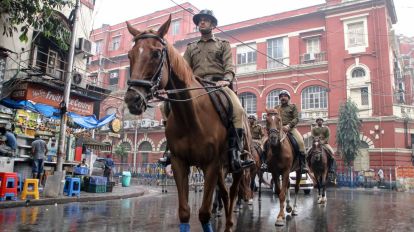In this photograph, we see a scene of a downtown city street featuring a procession of at least four men on brown horses. They are wearing brown military uniforms—comprising khaki pants, black boots, long-sleeve shirts, and caps—and are moving toward the camera. The day appears to be rainy, evidenced by the clear reflections of the riders and horses in the wet surface of the road.

In the background, a prominent three-story red brick building with numerous white-trimmed windows looms over the scene. To the left of the street, there's a more modern structure with a bustling market front. Here, people are seen shopping near a collection of variously colored items including a noticeable reddish newspaper machine, a yellow chair, and a blue chair, all separated by a light pole. Additional details include small stools or chairs by the street, adding to the dynamic urban atmosphere that contrasts with the unexpected presence of mounted men on horses.